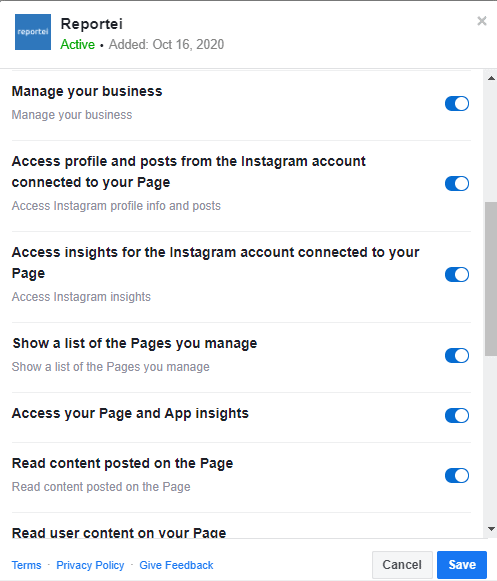The desktop screenshot features a predominantly white background with a detailed interface layout. In the top left corner, the company name "ReportAReportEI" is displayed prominently. Directly beneath this, the status "Active" is indicated in green text, separated by a dot from the note "Added October 16, 2020."

To the left of this information is a bluish square with the company initials "Report A." On the extreme top right is a small X mark used for closing the window. Below these elements, a series of listings are arranged, each with toggle buttons that are currently activated, signaled by their position to the right and a blue trail on the left.

The listings are as follows:
1. "Manage Your Business"
2. "Access Profile and Posts from the Instagram account connected to your page"
3. "Access Insights for the Instagram account connected to your page"
4. "Show a List of the Pages You Manage"
5. "Access Your Page and App Insights"
6. "Read Content Posted on the Page"
7. "Read User Content on Your Page"

A grayish scroll bar is placed centrally, equipped with up and down arrows at its top and bottom.

At the bottom left, several hyperlinks are displayed in blue text: "Terms," "Privacy Policy," and "Give Feedback." To their right are two buttons: a gray "Cancel" button and a blue "Save" button.